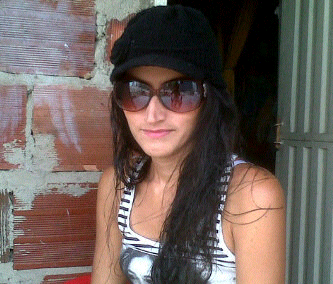In this image, a woman is sitting outside in front of an open white door, which reveals a dark interior behind her. To her left, there's a structure built from large bricks with visible mortar lines. She’s wearing a black hat and large, round, purple-tinted sunglasses, with a slight smile on her face. Her long, brown, slightly wavy hair drapes over her shoulder. She sports a white tank top with black lines along the shoulder straps and chest area. The tank top features a partial image of a woman's face, though only a small portion is visible.